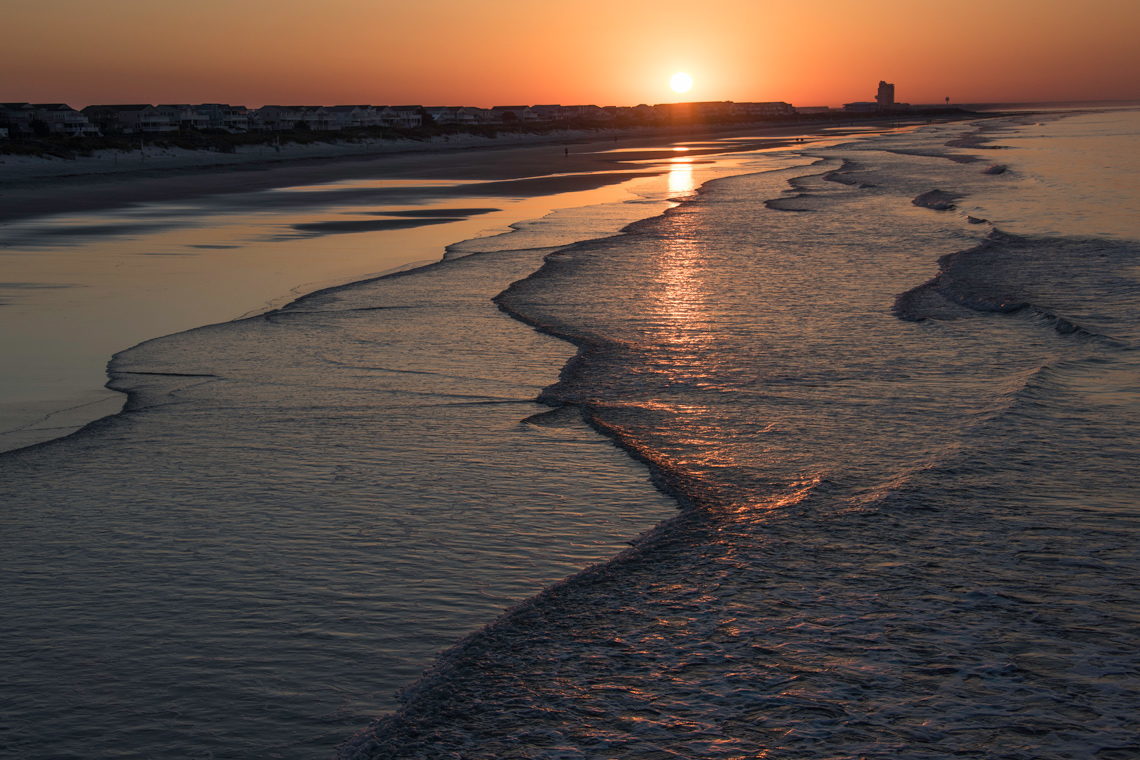In this high-quality photograph, we observe an enchanting beach town during the magical hour of sunset. The viewpoint is overhead, capturing the soft, methodical waves of the ocean gently caressing the shore. The coastline, lined with beach houses and perhaps small hotels, stretches off into the distance, where a single tall building stands far back, marking a less touristy atmosphere. 

The horizon is composed mainly of these residences, which are cast in shadow due to the setting sun. The sun, positioned slightly to the right of the center image, is beginning to dip below the horizon, casting a profound peach and orange glow throughout the sky. The sun's rays are beautifully reflected on the ocean's surface, enhancing its light blue ebb. Toward the left of the image, the horizon includes a pier or walkway ending in either a rock formation or a structure that adds to the scenic charm. There are no individuals or text in the image, allowing the serene beauty of the moment to take center stage. The rich gradient of colors transitions from light blue near the shore to deeper purples and pinks in the sky, creating a mesmerizing display that epitomizes the tranquil beauty of a coastal sunset.